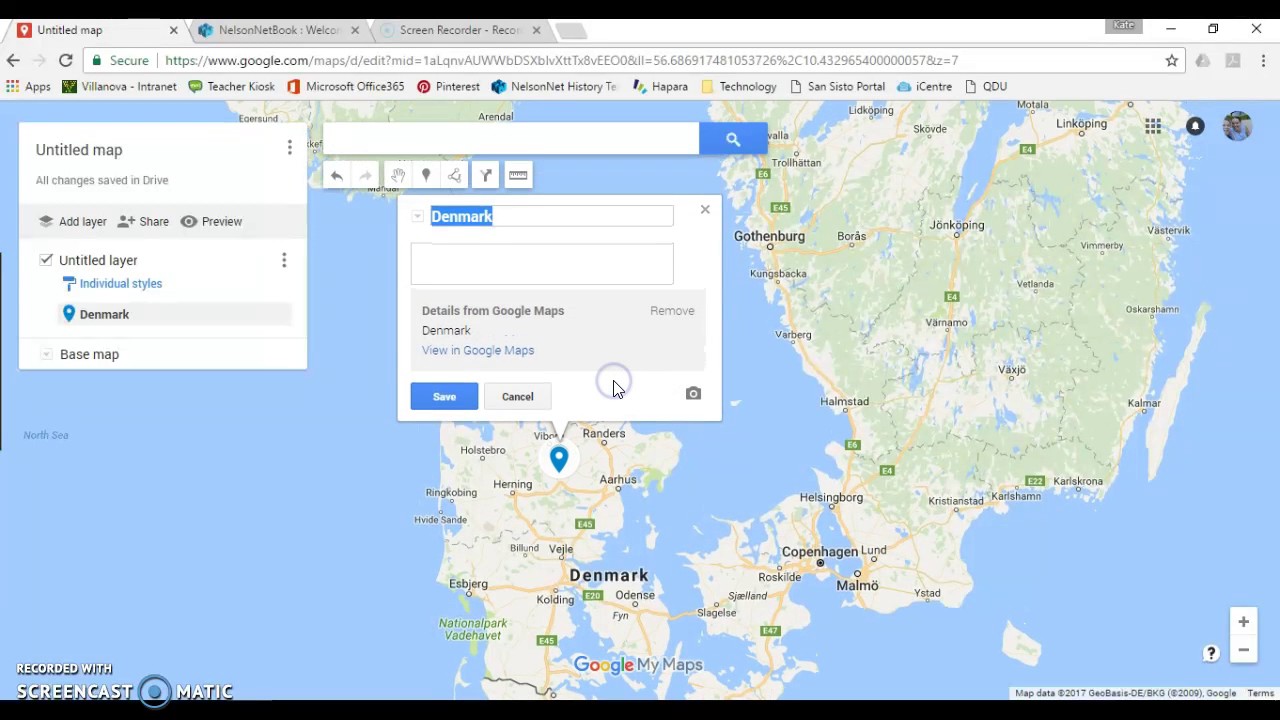The image is a screenshot from an older version of the Google Chrome web browser displayed on a desktop. The browser is showcasing a map of Denmark on a custom mapping tool. On the left side of the screen, there is a sidebar labeled "Unedited map" featuring various options and clickable icons, enabling the user to personalize and save their maps. A search bar is situated adjacent to this sidebar. Within the main display, multiple drop-down points are visible on the map, indicating areas of interest or customization.

A dialog box is open, allowing the user to name their map; it is currently titled "Denmark," with the name highlighted, suggesting a potential rename. Above the map and editing tools, the standard browser interface is visible, including the tab bar with three open tabs, the URL bar, navigation buttons (back, forward, refresh), and other typical browser elements. This overall setup indicates that the user is actively editing or creating a personalized map of Denmark using the browser-based tool.